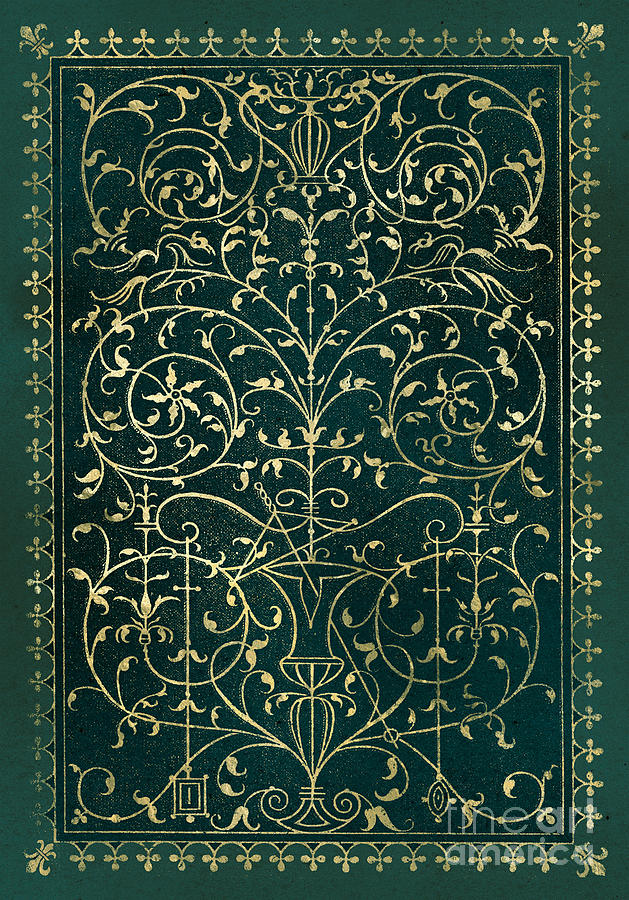The image depicts an ornate, possibly Turkish or oriental rug, measuring approximately 5 by 7 or 8 by 10 feet. It is displayed vertically and features a rich, deep forest green background with subtle gradations in color depth. The rug is bordered by a lighter green outer edge, typical of traditional oriental rugs. The intricate designs are rendered in gold thread or weaving, creating an elegant, symmetrical pattern reminiscent of antique book covers or fancy iron gatework. The gold pattern features six ornate spirals adorned with leaves and vines, along with vase-like elements at the top and bottom. There is also a unique triangular, kite-shaped formation subtly integrated into the design. Surrounding the central area, the border displays delicate fleur-de-lis motifs and straight lines, all maintaining a cohesive aesthetic. At the bottom of the image, the words "The Art America" are inscribed, adding a final touch to the overall composition.